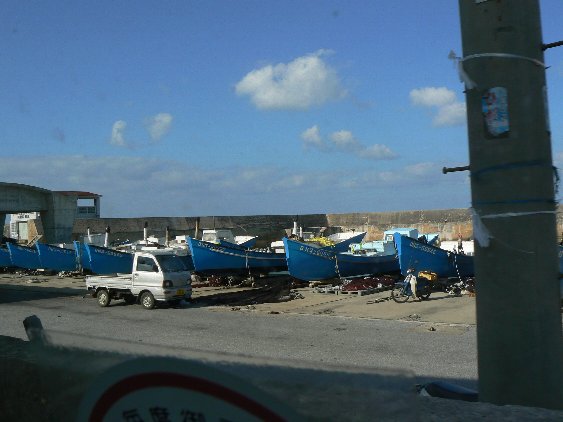This detailed color photograph appears to be taken in a shipyard in another country, showcasing a slightly run-down scene. The foreground features a large concrete pole on the right-hand side and a partially visible white sign with a red line, possibly written in Japanese or Chinese. Behind the sign, a one-lane road stretches, followed by the cab of a small silver flatbed truck. The standout feature of the image is a row of seven or eight large blue fishing boats lined up in front of a concrete wall. Some chains dangle from the boats. On the left side of the image lies a concrete building resembling a gray warehouse. The background is marked by a beautiful blue sky scattered with puffy white clouds. Additionally, on the right side, there’s a man in a white uniform riding a bicycle, adding a human element to the industrial setting.